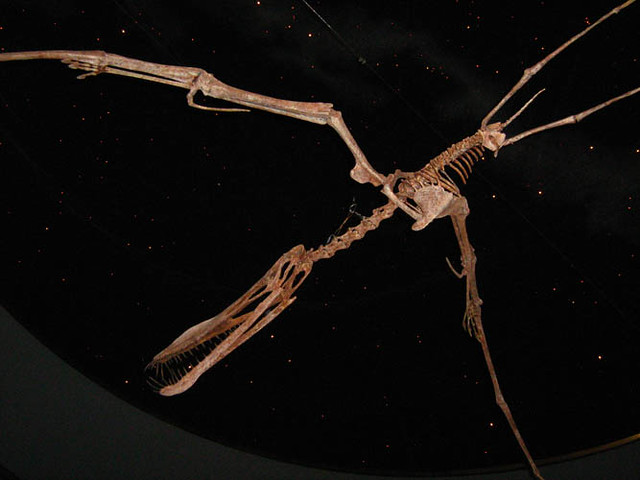The image shows a detailed, amber-toned skeleton suspended against a black background, potentially resembling that of a prehistoric creature or a large insect. The specimen, which exhibits characteristics like long antennas and an angular elongated head, has a thin body and wings that are spread wide, spanning from the top left to the bottom right corner of the frame. The wings, although skeletal, outline where fin or membrane-like material once was. The delicate structure includes a long neck, short body, tiny tail, and distinct legs. The scene is either taken at night or in a dark room, with the skeleton seemingly hanging near the ceiling, viewed from below, adding an almost eerie dimension to the setting. White specks in the background might indicate artificial lighting or possibly stars, emphasizing the stark silhouette of the skeleton against the dark backdrop.